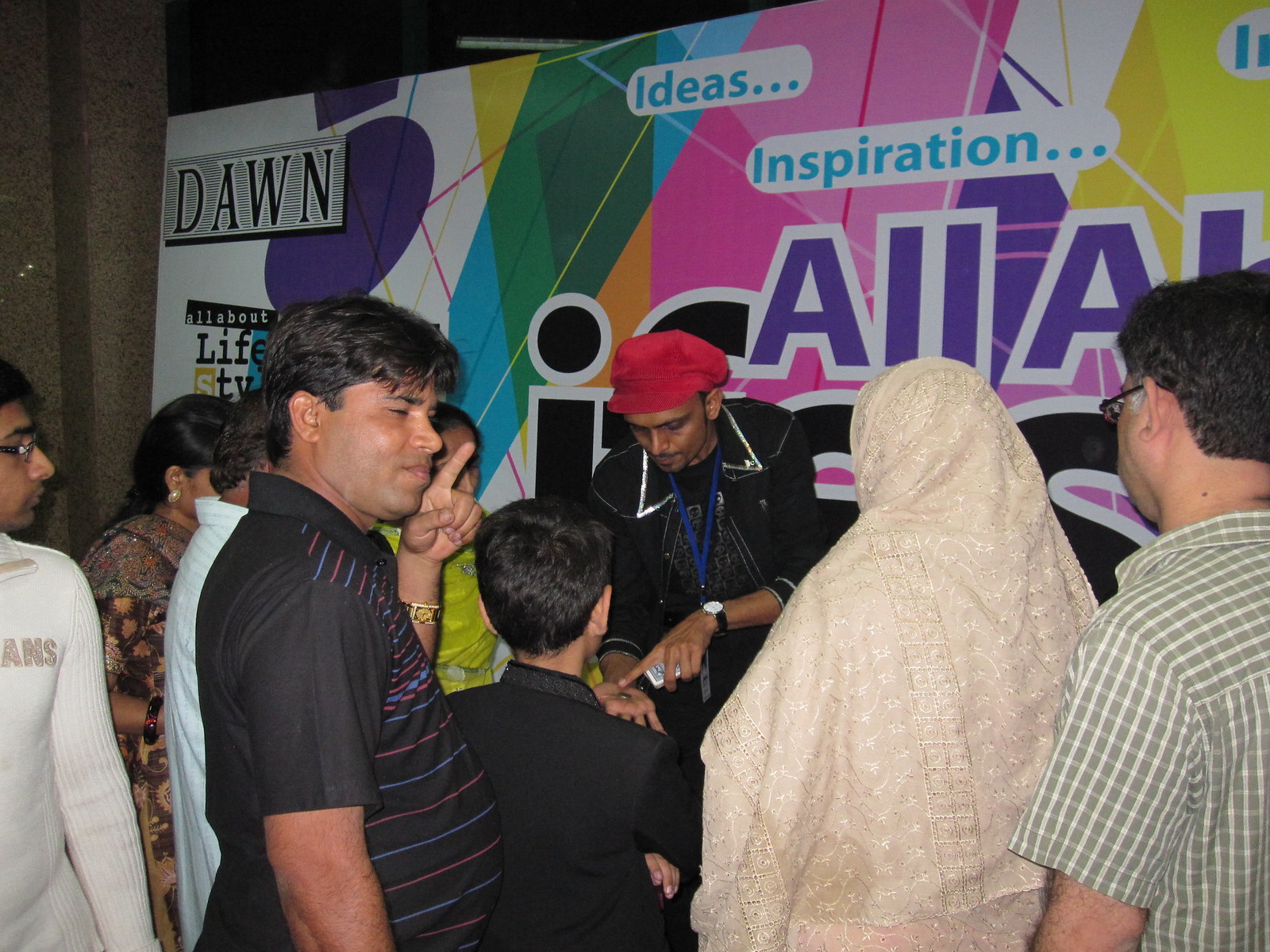A vibrant and colorful scene depicts several Indian people gathered at some sort of event, likely indoors given the dark lighting. The backdrop is a large, multi-colored banner adorned with geometric shapes in green, pink, yellow, orange, and more. The top left of the banner features the word "DAWN" in black letters, set against a black and white background. Below it, two white thought bubbles contain the words "ideas..." and "inspiration..." in light blue letters. There's also partially obscured purple text at the bottom. In front of this banner stands a man who appears to be performing a magic trick. He wears a red hat, black long-sleeved jacket with glittery edges on the collar, and a blue lanyard around his neck. He holds a deck of cards in one hand and points at a coin in his other hand's palm. Surrounding him, a crowd of captivated onlookers includes a woman with a white head shawl and a man in a black shirt with blue and red stripes, who is pointing upwards with his eyes closed. The scene hints at a lively and engaging performance.